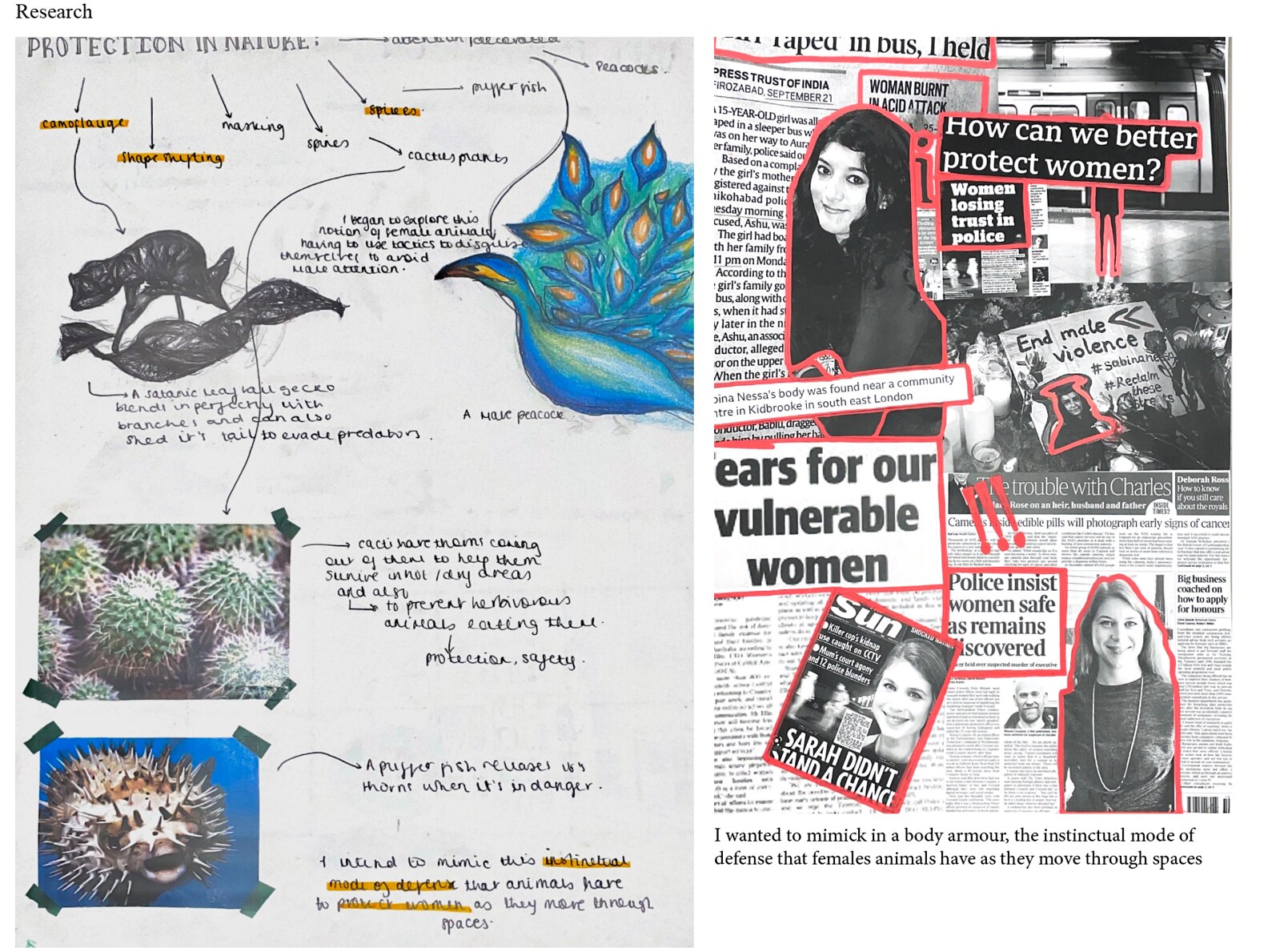The image appears to be a scanned two-page spread from a detailed research notebook, blending artistic and informative elements. The left page is rich with colorful hand-drawn illustrations and accompanying notations, emphasizing various animals and their natural defenses. A vividly colored peacock occupies a central space, annotated with informational arrows pointing to its distinct features. Other drawings include a creature, likely a charcoal or pencil sketch, shown running on tree branches, and a puffer fish accompanied by cacti images, all seemingly taped on but actually rendered with a stylized look. Each element is encircled by arrows and highlighted text providing detailed descriptions.

The right page presents a stark contrast with a collage of black-and-white newspaper clippings highlighted with bold red borders, focusing on societal issues related to women's safety. Headlines like "How can we better protect women," "Women losing trust in the police," and "Years for our vulnerable women" emphasize the theme of vulnerability and the need for better protection mechanisms. At the bottom, a thoughtful note reads, "I wanted to mimic in a body armor the instinctual mode of defense that female animals have as they move through spaces," drawing a parallel between the defense mechanisms of female animals and the societal need for protecting women. The entire page weaves together articles, images of women, and elements of defense strategies used by female animals, creating a powerful commentary on safety and protection.

Overall, the contrasting but interconnected pages combine vibrant, lifelike sketches of nature with sobering, monochromatic clippings, presenting a comprehensive study on the themes of protection and vulnerability in both the animal kingdom and human society.